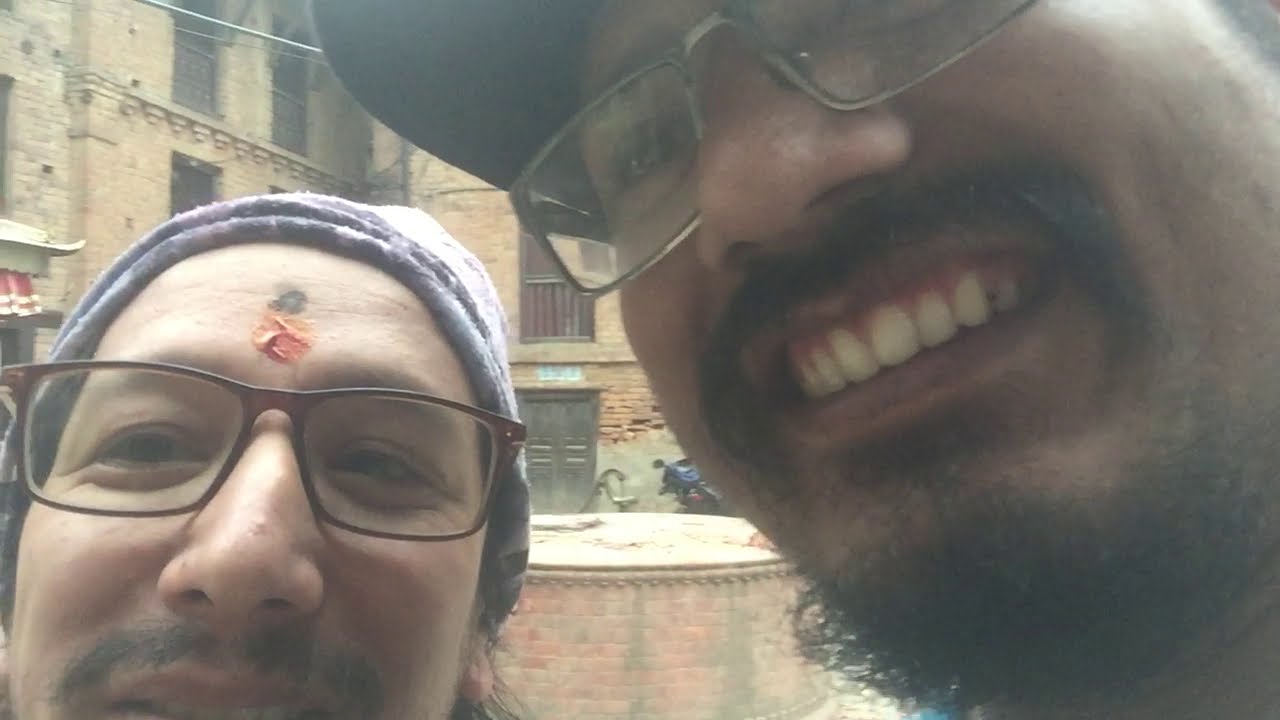In a close-up selfie, two men are smiling at the camera in what appears to be a historic brick plaza, possibly in the Middle East, with an old brick well or circular construction in the background. The man on the left, partially cropped from the bottom left of the image, has glasses, a thin mustache, and is wearing a purple sock cap. He also has distinct markings on his forehead: a small reddish paint mark followed by a black circular dot. The man on the right, more prominently in the image, is a glasses-wearing Caucasian with a beard, goatee, and a ball cap. Both are smiling, adding a warm, joyful atmosphere to the scene set against the backdrop of old brick structures.